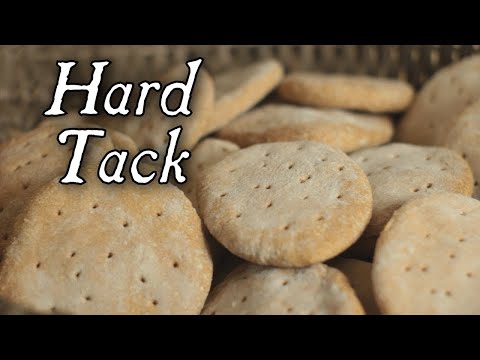The thumbnail image appears to be a still from a YouTube video, featuring a collection of light tan cookies, possibly hard tack or a similar type of biscuit. The cookies, distinctive with their multitude of tiny pin-sized holes, are stacked in a wicker basket that's either white or gray. The cookies themselves have a slightly whiter top compared to their darker edges, suggesting they are well-baked. The photo is framed by black bars at the top and bottom, giving it a cinematic look. In the top left corner, there's bold, white text with a drop shadow that reads "Hard Tack," written in partially capitalized letters (H and T capitalized), adding depth and emphasis to the image. The cookies are piled up, with some stacked higher in the background, creating a sense of abundance. The overall presentation suggests a focus on the baking or cooking process.